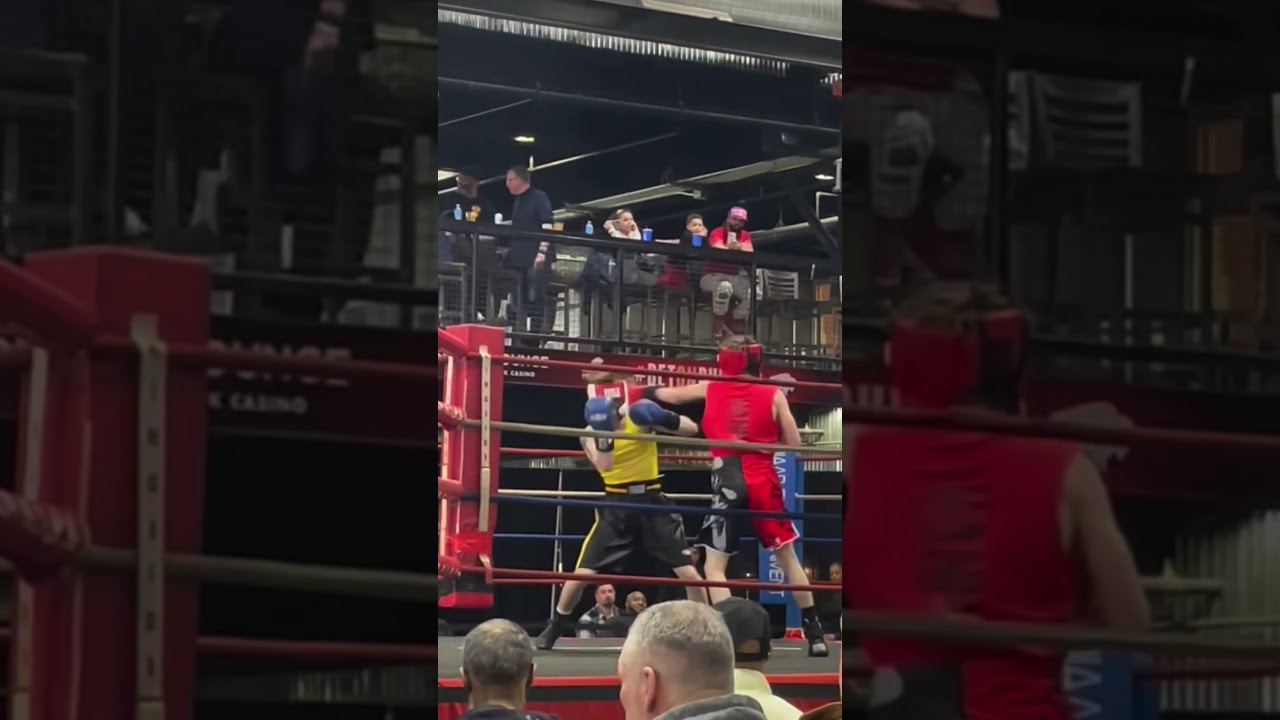This is a color photograph taken at a boxing match, featuring a creatively edited presentation. The central part of the image is the original, brightly lit section, framed by darker, enlarged, repeated portions of the same scene on the left and right sides. The boxing ring has a black floor and is bordered by red skirting with red, white, and blue ropes. Prominent red corner posts add to the vibrant setup.

In the ring are two boxers: one with his back towards the camera, wearing red headgear, a red sleeveless shirt, and red and black shorts. His opponent, mostly obscured by defensive arm positions, faces him while donning white headgear, blue boxing gloves, a yellow sleeveless shirt, and black shorts with yellow stripes. The ring action is intense, with the boxer in red in mid-punch, aiming at his opponent.

In the foreground, from a ground-level perspective, we see the backs of three spectators. Above them, a second story or balcony level houses more onlookers, some sitting and others standing. This upper level has a black metallic-looking overhang and attendees appear to be engaged in eating and drinking, with visible blue cups and bottles. The creative repetition of the image frames the energetic scene within a darker border, emphasizing the central, lit-up action.